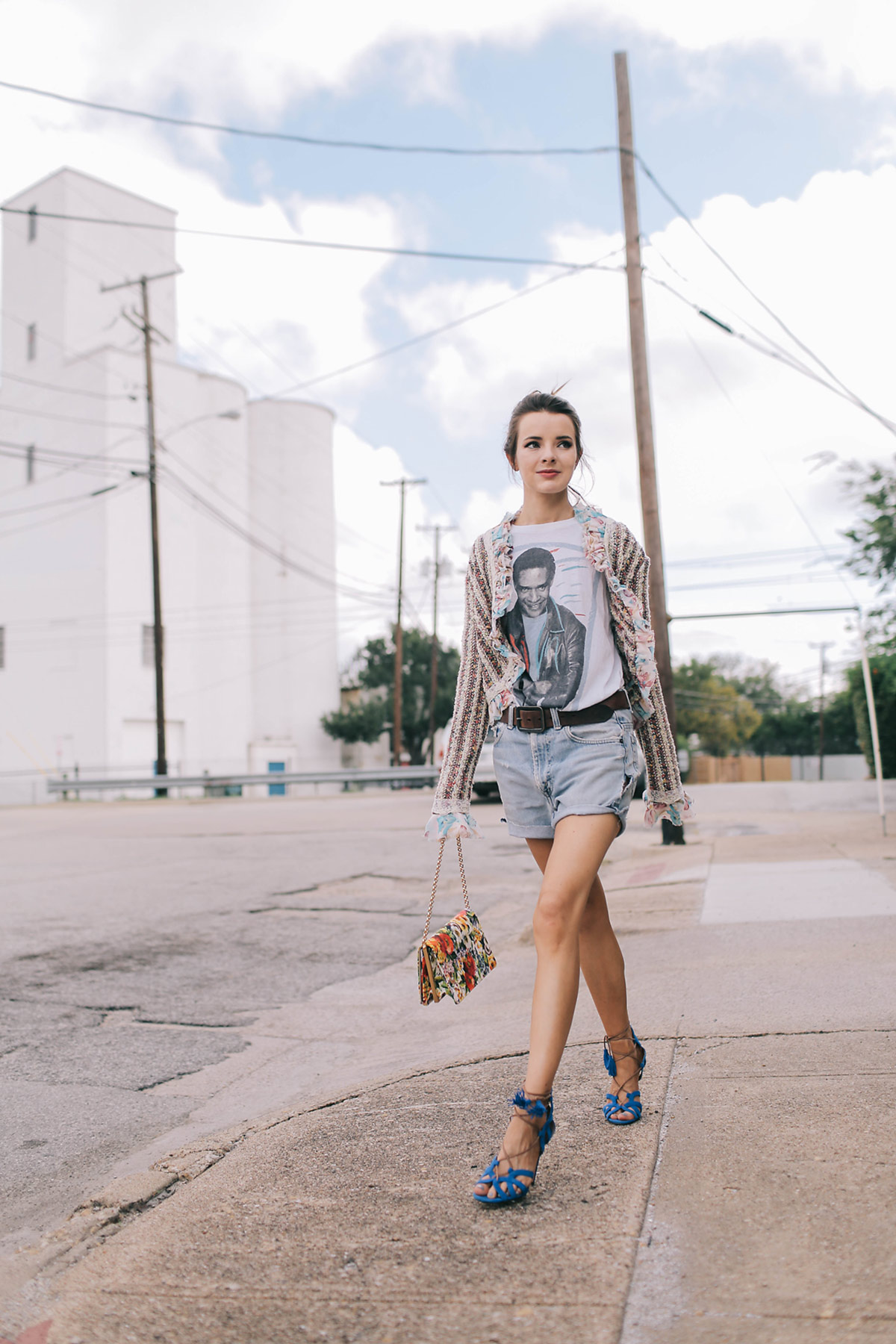The photograph captures a confident young woman, likely in her early 20s, walking down a street that appears to be in an industrial area. She is impeccably dressed in a stylish ensemble that includes beautiful blue high heels, light blue denim shorts secured with a brown leather belt, and a graphic tee featuring an indistinct person, tucked into her shorts. Over her t-shirt, she wears a cardigan with long sleeves, suggesting a nuanced blend of casual and sophisticated fashion. Her brown hair is swept up, possibly in a bun or ponytail, adding to her poised appearance. A small, colorful purse adorned with floral patterns dangles from one of her hands, which are hidden by the long sleeves. In the background, the setting is characterized by slanted telephone poles with electric wires extending from both sides, a vast white building, and part of a tree. The sky overhead is cloudy, casting a diffused light on the scene below, emphasizing her as the focal point of this fashion-oriented photograph.